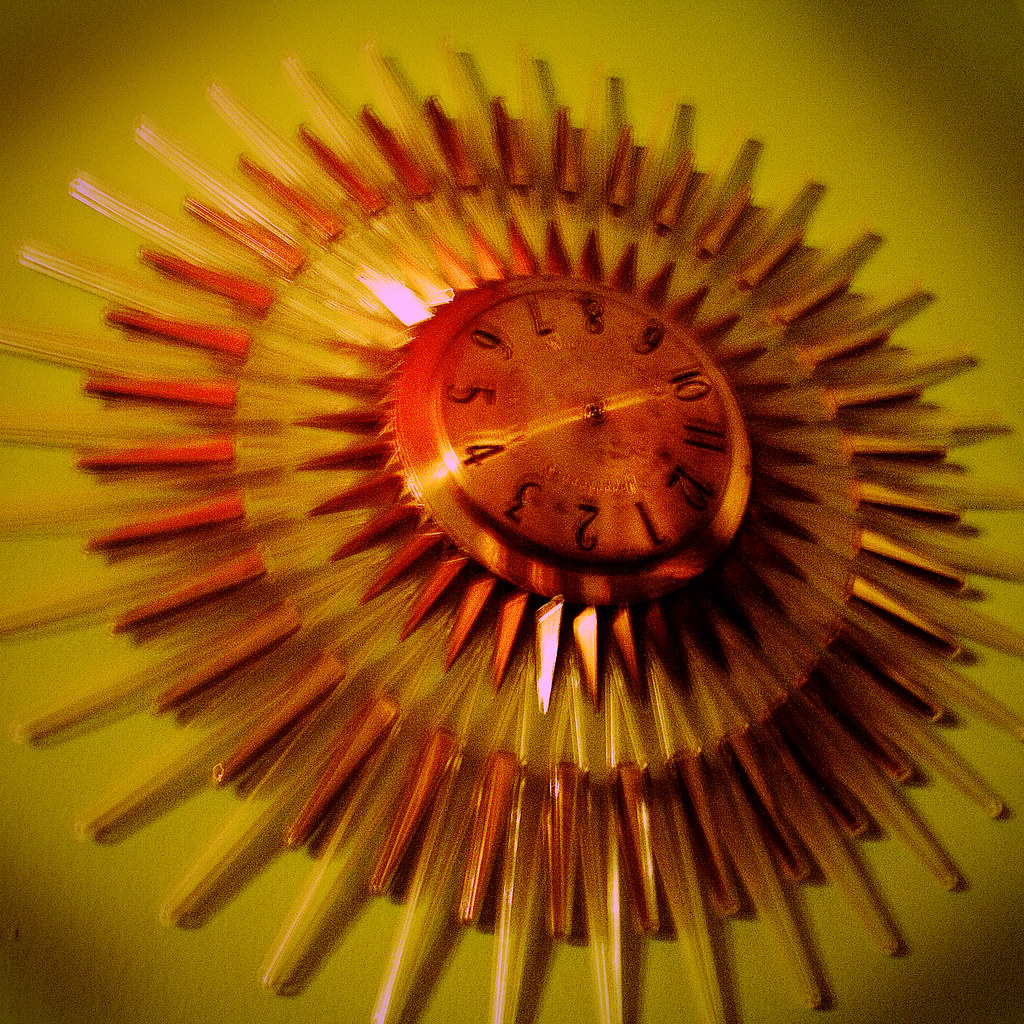This square color photograph captures a dramatic, mid-century sunburst wall clock set against a lime greenish-yellow background. The photo is uniquely rotated so that the number 12 is pointed downwards to the right. The central face of the clock is a vivid orangey-red with black numerals, though the hands of the clock are absent or unclear, possibly due to light reflections. The clock design features multiple layers of radiating spikes: an inner layer of orange metal spikes, followed by a translucent layer, and then a final outer layer of yellowish plastic spikes, all contributing to its sun-like appearance. The unusual lighting casts a red hue over the clock, creating a surreal effect, while the darker shadows at the corners of the photograph add depth and contrast. Overall, the image is vibrant and detailed, showcasing the clock as a radiant centerpiece against a compelling backdrop.